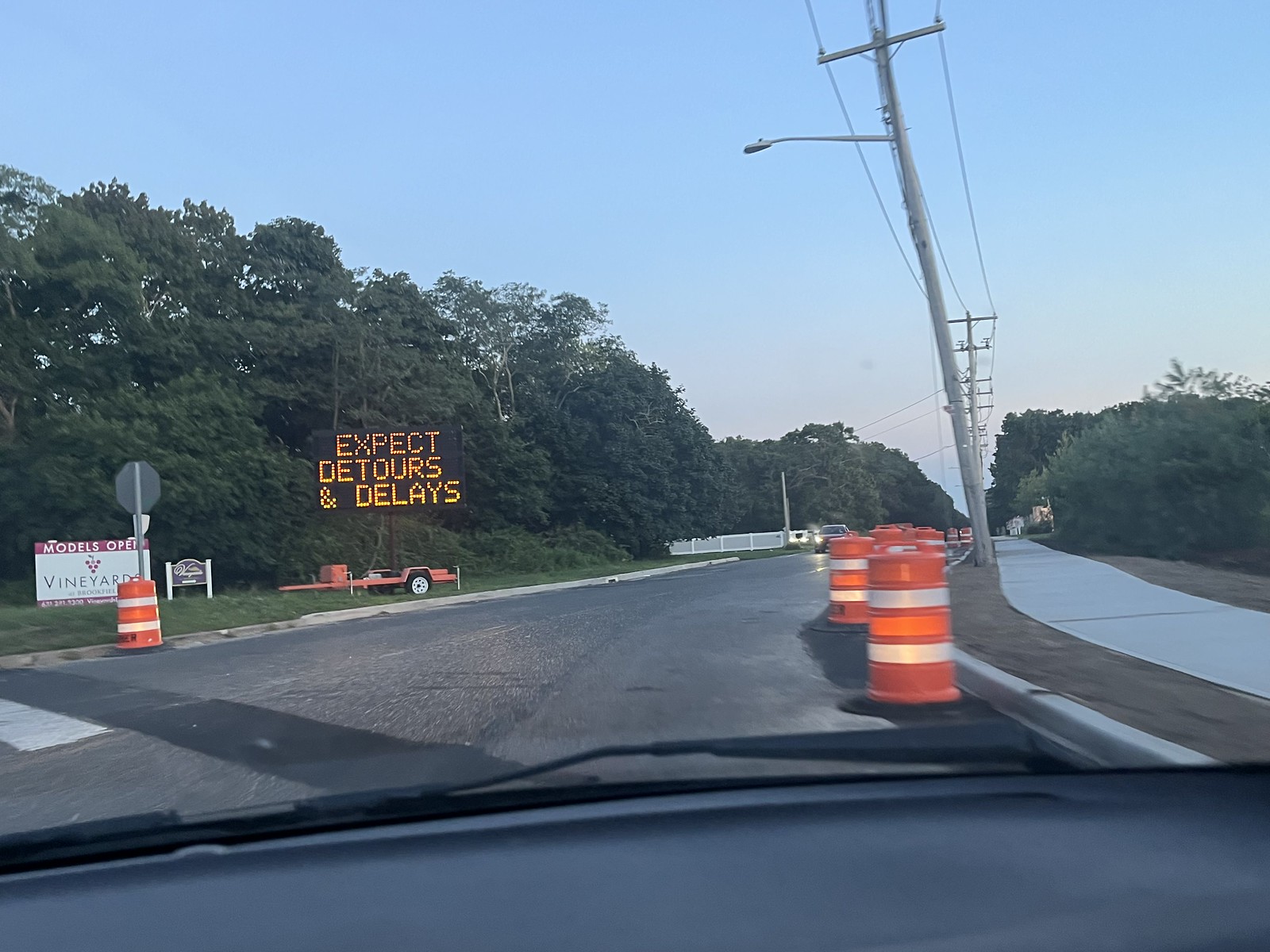This detailed photograph, taken from inside a dark gray vehicle, captures an intricate scene of a construction zone. The vehicle's black dashboard and windshield wipers frame a view of a road under repair, characterized by dark gray asphalt with numerous light and dark gray tar patches. On the right-hand side of the road, a freshly poured, pristine light gray sidewalk is bordered by bare brown dirt, indicative of recent installation. A row of orange construction barrels with white stripes lines the right side of the road, accompanied by a single barrel on the left, positioned in front of a stop sign and additional signs. One prominent sign, a large electronic LED construction trailer, displays "Expect Detours and Delays" in bright orange. Nearby, an advertisement for "Vineyards" includes a drawing of red grapes, signaling model homes. The left side of the road features a long line of lush dark green trees and a white fence, interspersed with occasional bushes. This vibrant snapshot is completed by the bright blue sky, dotted with clouds, and a few oncoming cars, suggesting a busy day despite the absence of visible construction workers.